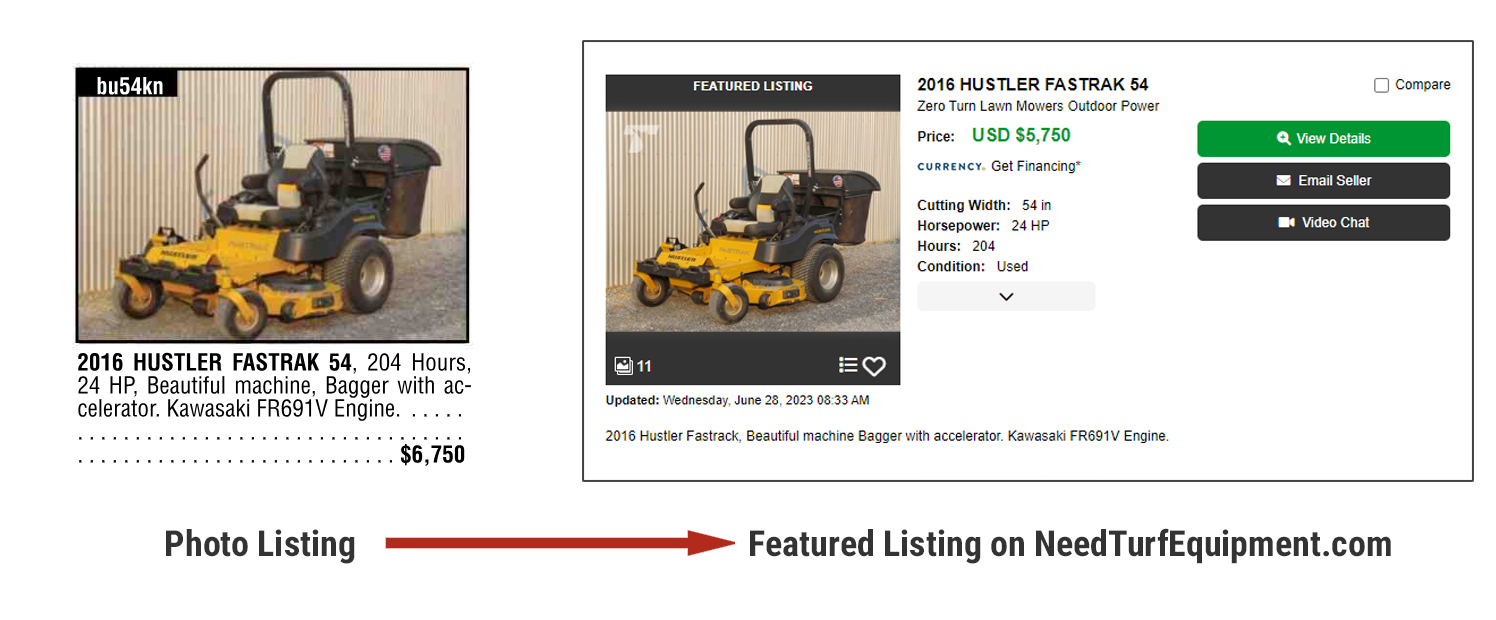Screenshot of a webpage featuring a listing for a 2016 Hustler Fast Track lawnmower.

On the left-hand side, there's an image of the lawnmower set against a black background. The lawnmower is yellow and positioned on a gravel surface, with a wall displaying vertical striping behind it. In the top left corner of the image, a black horizontal box displays the text "BU54KN" in white.

Below the photo, detailed information about the lawnmower is presented: 
- Model: 2016 Hustler Fast Track
- Cutting width: 54 inches
- Hours used: 204
- Horsepower: 24 HP
- Features: beautiful machine, bagger with accelerator, Kawasaki FR691V engine
- Price: $6,750 USD

On the right-hand side of the screenshot, there is a white horizontal box with a black border. The same image from the left is repeated within this box, labeled as a "featured listing." Additional details include an update timestamp: Wednesday, June 28, 2023, at 8:33 a.m. Repeating the product information, it confirms:
- Model: 2016 Hustler Fast Track, zero-turn lawnmower
- Category: Outdoor Power Equipment
- Price: $5,750 USD
- Financing options available
- Technical specifications: Cutting width of 54 inches, 24 HP, 204 hours used, condition marked as "used."